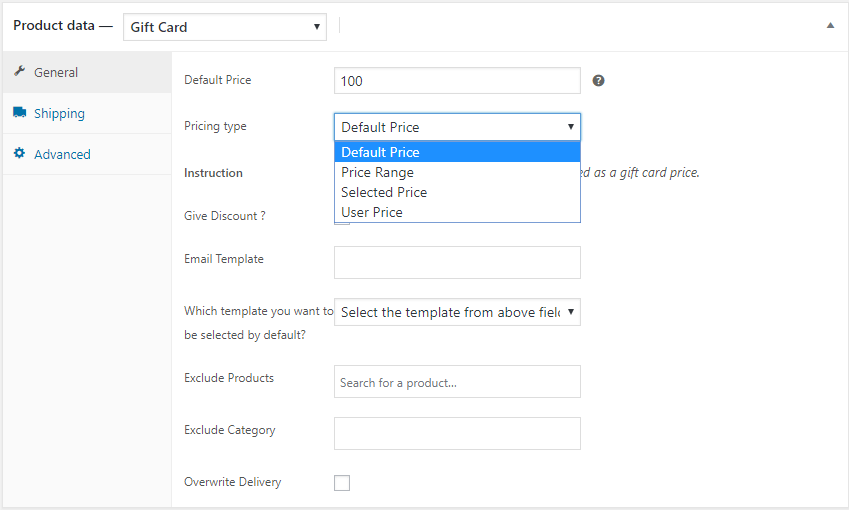A detailed, cleaned-up descriptive caption for the image could be:

"The image displays an online interface for managing product data, with a user-friendly layout consisting of several sections. In the top left corner, the background is white, which contrasts with the adjacent black section labeled 'Gift Card.' 

To the right, there is a vertical gray column with the following categories listed in descending order: 'General' in gray, 'Shipping' in blue, and 'Advanced' in blue. Adjacent to this gray column, another section with a white background contains various settings and options for the gift card. 

Within this section, the following labels are in black text: 'Default Pricing Type,' 'Instructions,' 'Give Discount?' (with a question mark), 'Email Template,' 'Which template you want to be selected by default?' (including a question mark), 'Exclude Products,' 'Exclude Categories,' 'Overwrite Delivery.' Each option is followed by a corresponding input box.

Following these settings, the next column answers the categories with specific configurations. The first field displays '100' as the selected default price, highlighted in blue. However, the visibility of the discount options is obscured by a scroll tab showing multiple pricing types: 'Default Price,' 'Price Range,' 'Not Selected Price,' and 'User Price.' The 'Email Template' field is currently empty, with a hint text: 'Selected template from above field,' and an adjacent prompt for searching a product.

Further details in this section are partially obstructed, but visible text includes 'ED' (possibly part of a word) and 'as a Gift Card Price.' This segment concludes with the default price of the gift card set to $100, although some content is hidden by overlapping interface elements."